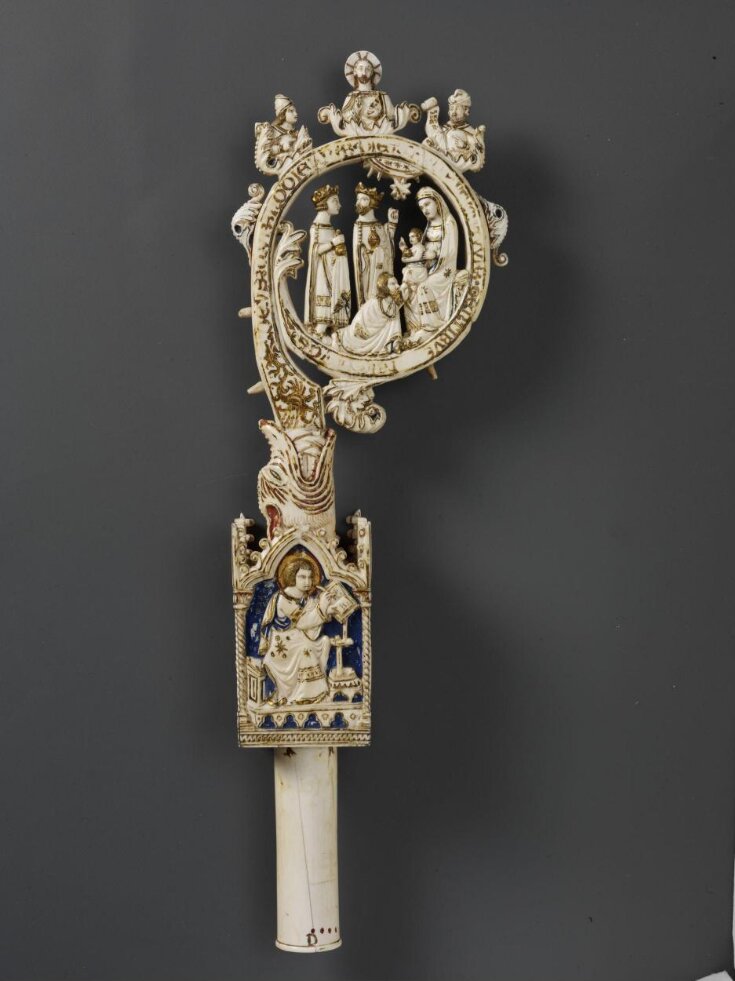This close-up image showcases an intricately designed artifact with a strong religious and mystical iconography, suggesting a possible Christian origin. The object, resembling a golden rod or staff adorned with black and brown accents, features detailed sculptural elements that give it an ornate, almost Tartarian, old-world charm. Central to the design are figures that appear to include Mary and three disciples, topped by a meditative figure resembling Jesus. The stem of the artifact includes sections with a blue background, depicting a woman seemingly inscribing scripture into a book. Additionally, the object bears images of kings and people bowing, adding to its spiritual and historical narrative.